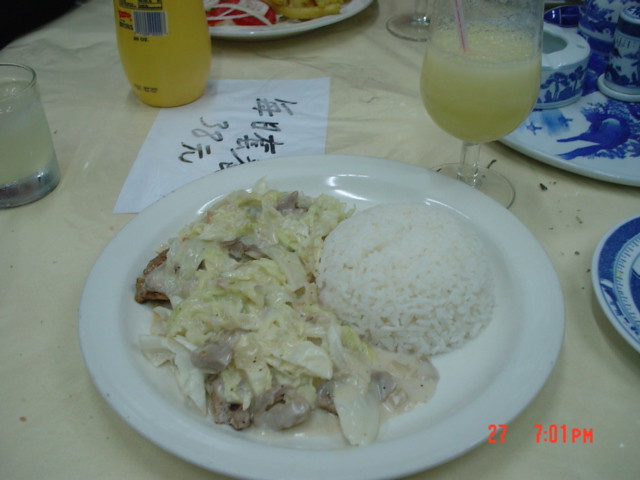This color photograph, taken indoors, captures a dining scene at a Chinese restaurant. In the lower right-hand corner, there is a red date and time stamp reading "27 7.01pm." The table is covered with a yellow cloth and adorned with blue and blue-and-white plates featuring intricate designs. At the center of the table is a plain white plate holding a generous scoop of white rice beside a beige-yellowish dish of meat and cabbage.

To the left of the plate lies a white piece of paper containing Asian writing, partially obscured by a yellow can. Two glasses of yellowish or orangish mixed drinks with red straws are also present—one behind the plate and another further to the left. This detailed setting invites you to delve into the intricate and colorful elements of an authentic dining experience.